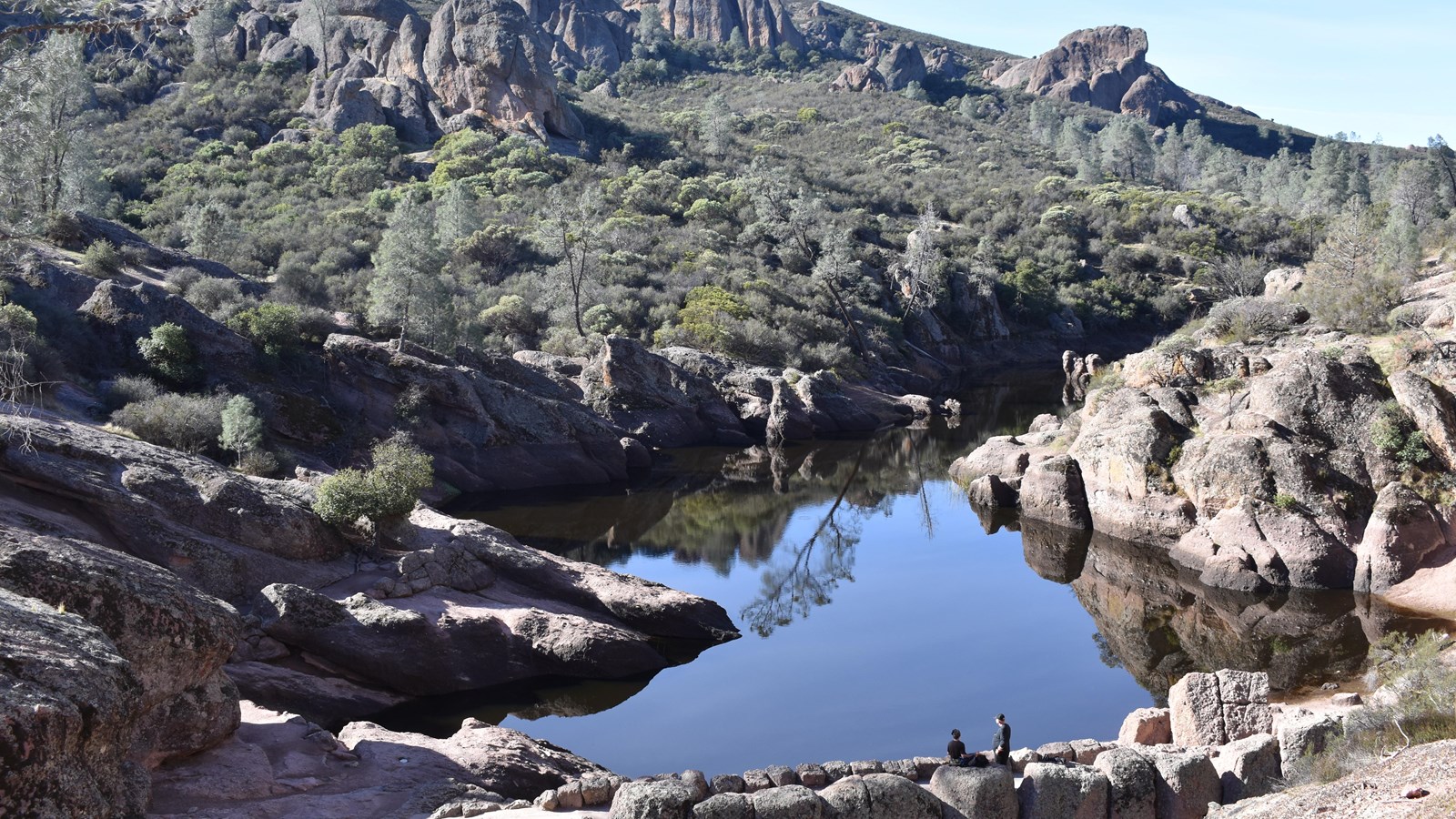The photograph captures a serene outdoor setting dominated by a small lake or pond cradled amidst rugged rock formations and a mountainous backdrop. At the top of the image, there's a glimpse of pale blue sky, suggesting clear weather. Descending from the upper right to the left is a majestic rock-studded mountain range. Below this, the terrain transitions into a more gentle, green-inclined cliff decorated with scattered trees and bushes. In the middle of the picture, the blue water of the lake reflects the sunlight, surrounded by grayish-white rocks that curve around it in a circular formation. In the foreground, at the bottom center, two small figures appear to be conversing while seated on one of the rocks. Their exact identities are indiscernible due to the distance. The lower portion of the image is peppered with additional rock formations that enhance the rugged, natural beauty of the scene, illuminated by the warm sunlight casting shadows and reflections on the water surface. The overall palette includes earth tones of brown and green, punctuated by the blues of the sky and water, along with hints of gray and black from the rocks.